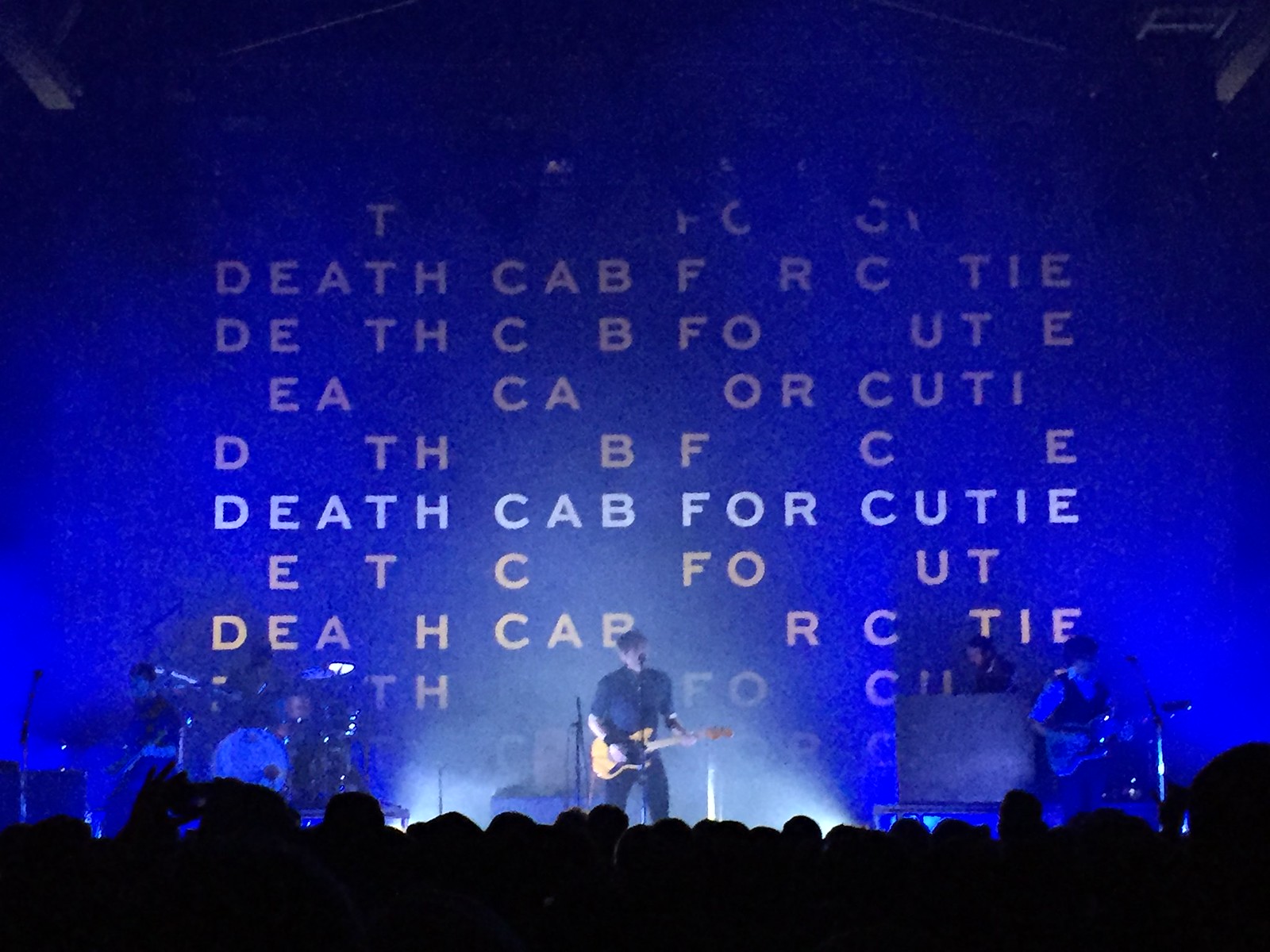This photograph captures a live concert performance by the band Death Cab for Cutie. The stage is enveloped in a hazy atmosphere, likely from a fog machine, giving the image a surreal, cutout appearance. The blue-hued background prominently features the band's name, "Death Cab for Cutie," in white letters, with parts of the text scattered above and below the central phrase. On stage, the band members are illuminated by spotlights: a drummer to the left, a keyboard player behind, a guitarist to the right, and the lead singer center stage, strumming a guitar and singing into a microphone. The bottom portion of the image shows the audience as dark silhouettes, with the outline of their heads tightly packed together. A concert-goer on the left is holding up a phone, capturing the electrifying moment.